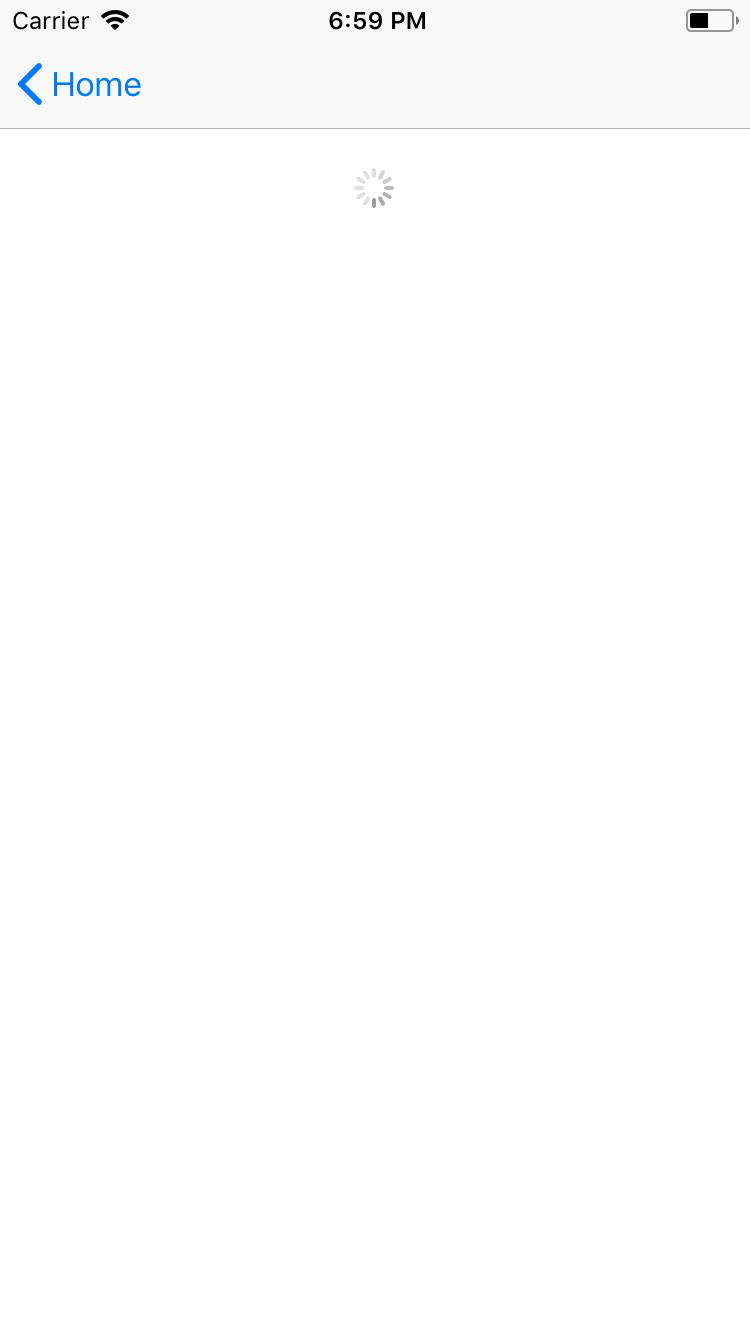A tablet screen is displayed with minimal information. At the top left, there are signal bars and Wi-Fi indicators, suggesting a connected device. The time, shown in the center at 6:59 p.m., is flanked by a half-full battery icon on the top right. The screen's main display area is predominantly white, save for a loading symbol—a circular icon in shades of gray—indicating the page is still loading, with only about a tenth of the page loaded. The bottom portion of the screen features a navigation bar, with a left arrow and a blue-highlighted 'home' icon on the left side, separated by a thin light-gray line. The overall color palette of the screen includes black, gray, blue, and white, emphasizing its minimal and functional aesthetic.